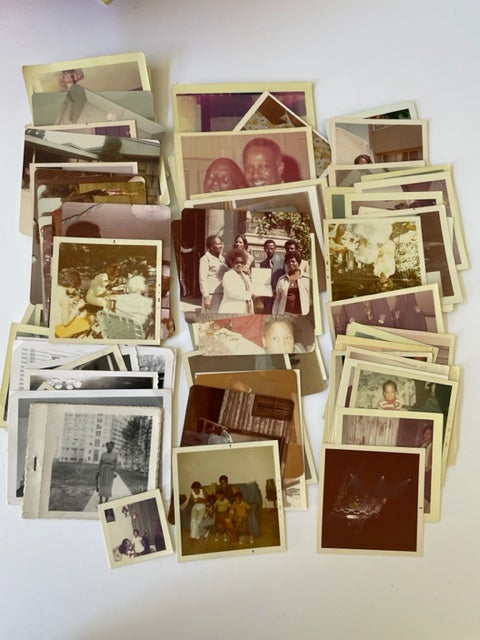The image captures a collection of approximately 60 to 100 vintage photographs scattered across a white or whitish-gray surface, arranged loosely into three stacks that fan out and overlap like a deck of cards. These photographs, primarily depicting African-American individuals and family moments, range in age from the 1940s to the 1970s, with some appearing as aged as the 1980s. The photos show signs of wear and fading, with many possessing the classic white or beige borders typical of that era's Polaroid prints.

Among the visible photos, a prominent one in the bottom middle showcases a family—a man, a woman, and three small children—seated on a blue couch. Another significant photo in the middle features five African-Americans, with one holding up a plaque, suggesting a moment of recognition or celebration. To the left of this, a smaller image shows a child, while above this arrangement, a black-and-white photo captures a woman in a long dress, standing in front of a tall building.

Scattered among these highlighted images are various other snapshots portraying intimate family scenes, such as another duo of older black men smiling, couples, and individual portraits. Some photos show single individuals, while others capture group scenes, some possibly post-church gatherings or similar events. The collection overall paints a poignant picture of familial love and history, preserved through the tradition of physical photographs.